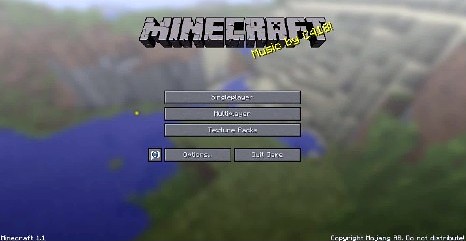The image is a horizontally rectangular screen capture from a video game, specifically from the start or menu screen of "Minecraft." The background is artistically blurred, presenting various colors in different corners: dark blue in the lower left, green in the lower right, gray in the upper right, and a mix of brown and green in the upper left. Prominently displayed in the center, the word "Minecraft" appears in a gray, brick-like texture. Crosscutting diagonally from the lower left to the upper right over the letters "F" and "T" of "Minecraft," it reads "Music By," followed by what seems to be the text "B4L8." In the center of the image, three horizontally rectangular menu buttons stack vertically. Below these buttons, there are two shorter, horizontally-aligned rectangular buttons positioned side by side.